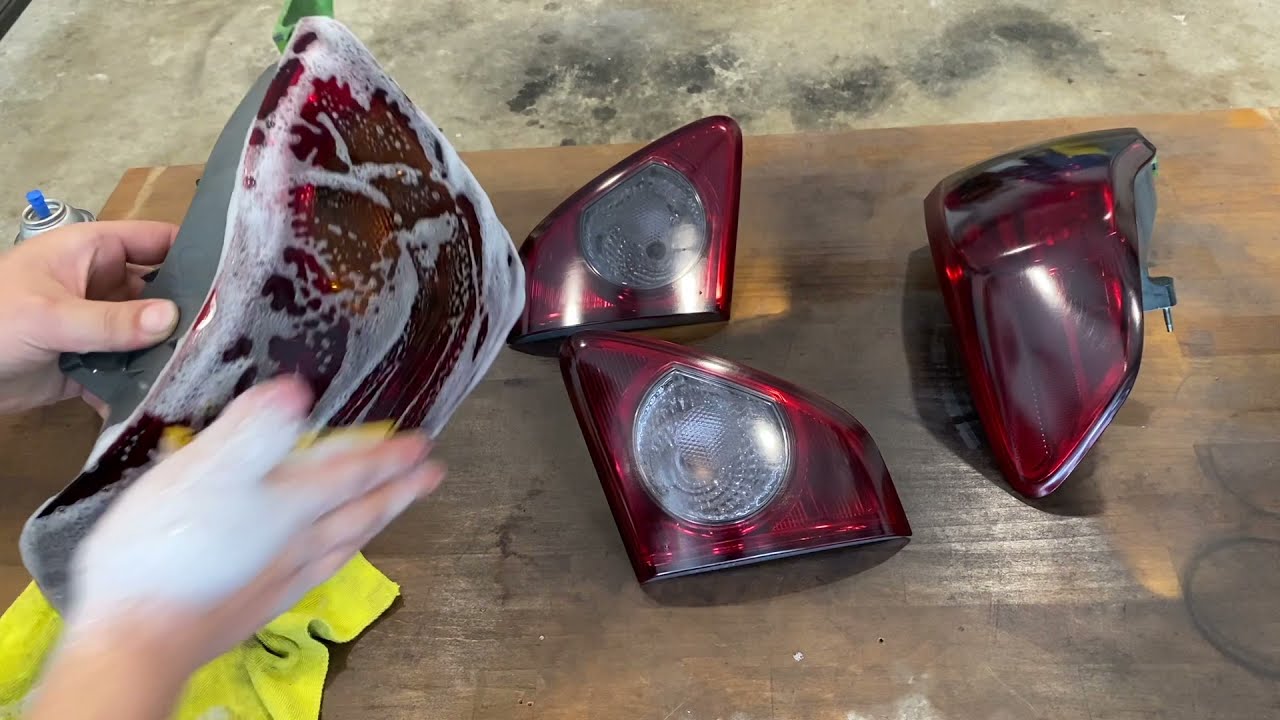The image shows a close-up scene of three triangular-shaped vehicle taillights with red interiors and silver bulbs, placed on a brown wooden board set on a gray, slightly grimy concrete floor. The taillights are shiny and reflect light well. On the left side, a pair of light-skinned human hands are holding the cover of another taillight, diligently scrubbing it with a small brush. The cover and brush are covered in white soap suds. Below the hands, on the wooden board, lies a yellow cloth, and near it, there is a spray can. The scene appears to be part of a demonstration on how to clean and polish taillights.